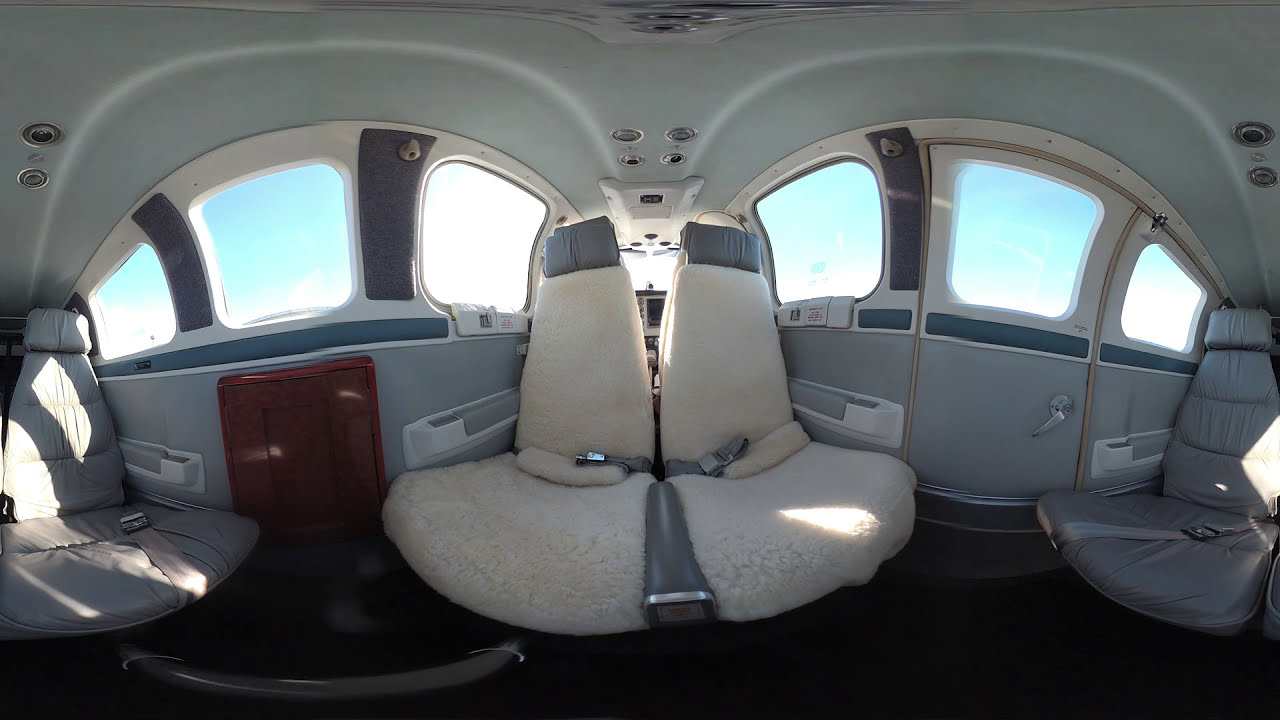This image depicts the luxurious interior of an airplane, likely the first-class section on a private jet or a high-end commercial airliner. Dominated by a sophisticated palette of white, light gray, and beige, the space exudes an aura of elegance and comfort. Central to the image are two plush, white seats in the middle, outfitted with gray headrests and seatbelts, showcasing a unique design where the top is slim and the bottom broadens out like a triangle. These seats, as well as additional pairs to the right and left, are clearly designed for premium comfort, intended for affluent passengers.

On both the left and right sides of the cabin, there are arches adorned with three windows each, through which blue skies and white clouds are visible, confirming that the airplane is in flight. Overhead, individual lights and ventilation vents are present, adding to the in-flight conveniences one would expect. The floor contrasts sharply with the light tones above, being almost pitch black, which further accentuates the immaculate cleanliness and modern aesthetic of the space.

The overall impression is one of pristine readiness—an unoccupied, spotless environment prepared for its next set of discerning travelers.